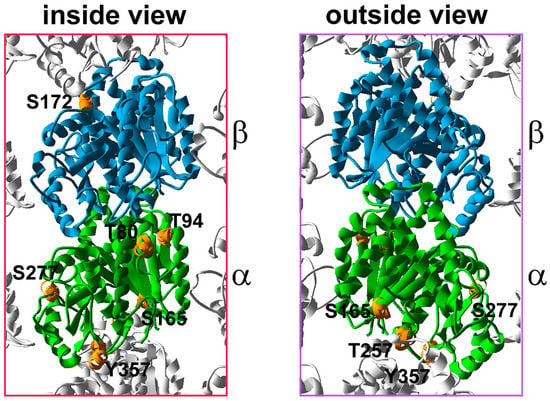The image features two scientific illustrations on a white background, labeled "inside view" on the left and "outside view" on the right. Both illustrations depict ribbon-like structures in blue and green, resembling molecular or atomic diagrams, with small golden nodules interspersed throughout. The blue ribbons are marked with a beta symbol (β) and the green ones with a lowercase sigma (σ), each accompanied by numerical labels such as S172, S165, and T94. Additional annotations include Y357 and S277. The "inside view" illustration is outlined in orange, while the "outside view" is outlined in purple. Surrounding the main structures are gray, similarly-shaped objects, and the overall arrangement suggests a biological or educational focus, potentially related to DNA or protein structures.